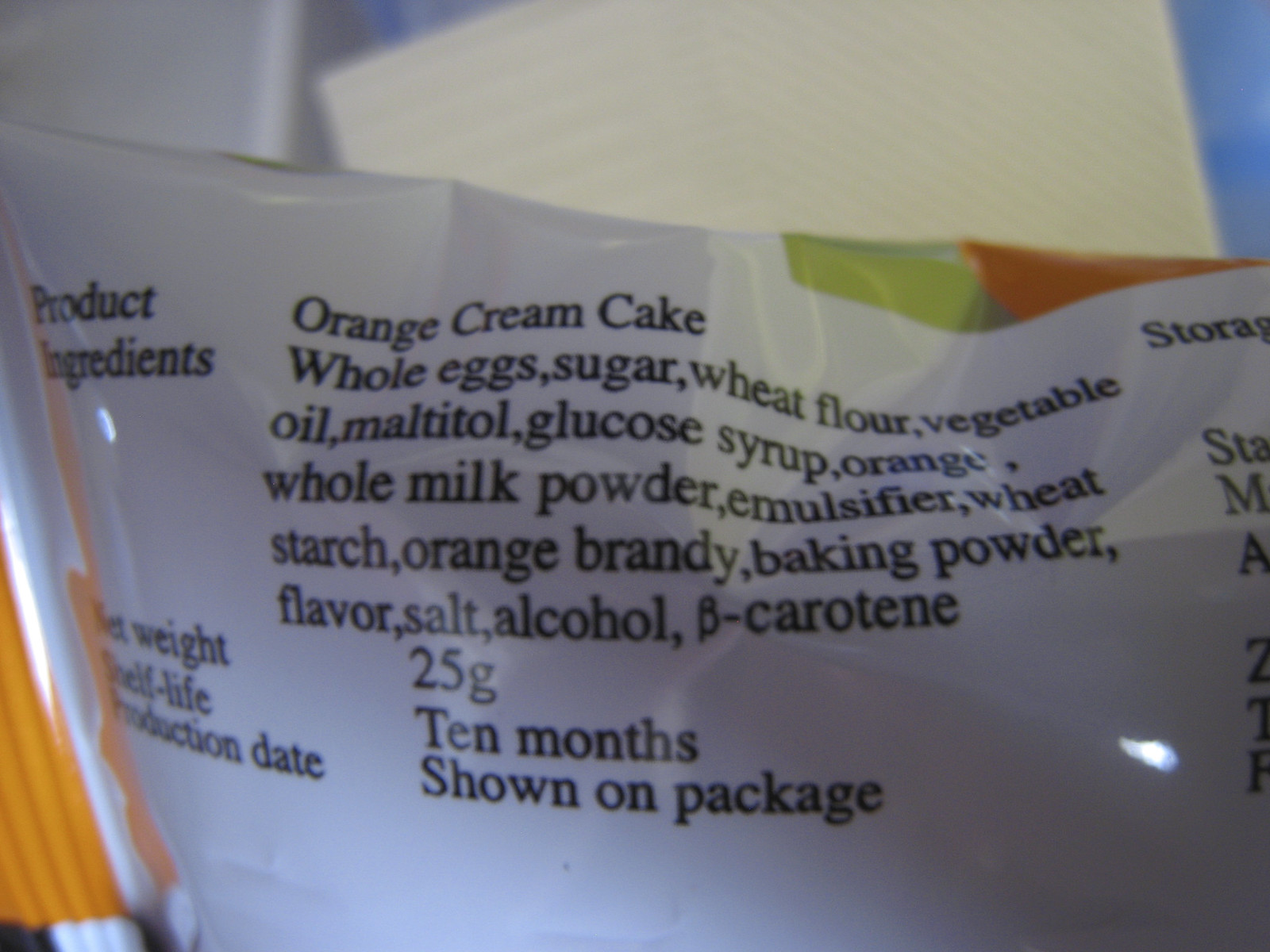The image showcases the back of a plastic bag containing an Orange Cream Cake. The packaging prominently displays the list of ingredients, which include whole eggs, alcohol, and salt, amongst others. Detailed storage instructions are provided, along with the information that the product has a shelf life of 10 months and a net weight of 2.5 grams. The production date is indicated on the package itself. There is a faint, light-colored image that appears predominantly white with a hint of blue on one end. The bag rests atop a paper towel on a blue countertop.